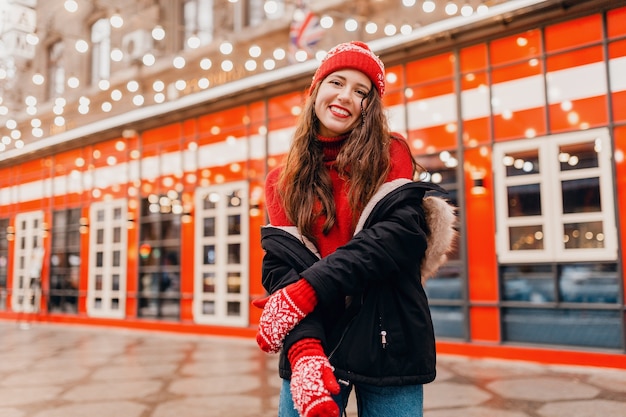This vibrant and colorful image captures a smiling woman standing on a wet sidewalk, hinting at recent rain or melting snow. She is poised in front of a striking orange-red building, adorned with white-trimmed windows and red trim. Strings of gold and white bistro lights drape across the building's facade, adding a festive touch. The building, possibly a large restaurant, bar, or entertainment center, features blue elements that may be interior decor visible through the windows.

The focus of the image is the woman herself, who stands out vividly against the background. She wears a matching ensemble of red—a beanie cap, a sweater, and mittens adorned with white snowflake-style accents. Her long dark hair cascades well past her shoulders. Over her outfit, she has a black, furry hooded coat, which hangs stylishly and slouches off her shoulders, adding a casual yet chic flair. Her jeans, red lipstick, and lightly flirtatious head tilt to one side enhance her playful yet cozy winter look. She gazes directly at the camera, her smile wide and inviting.